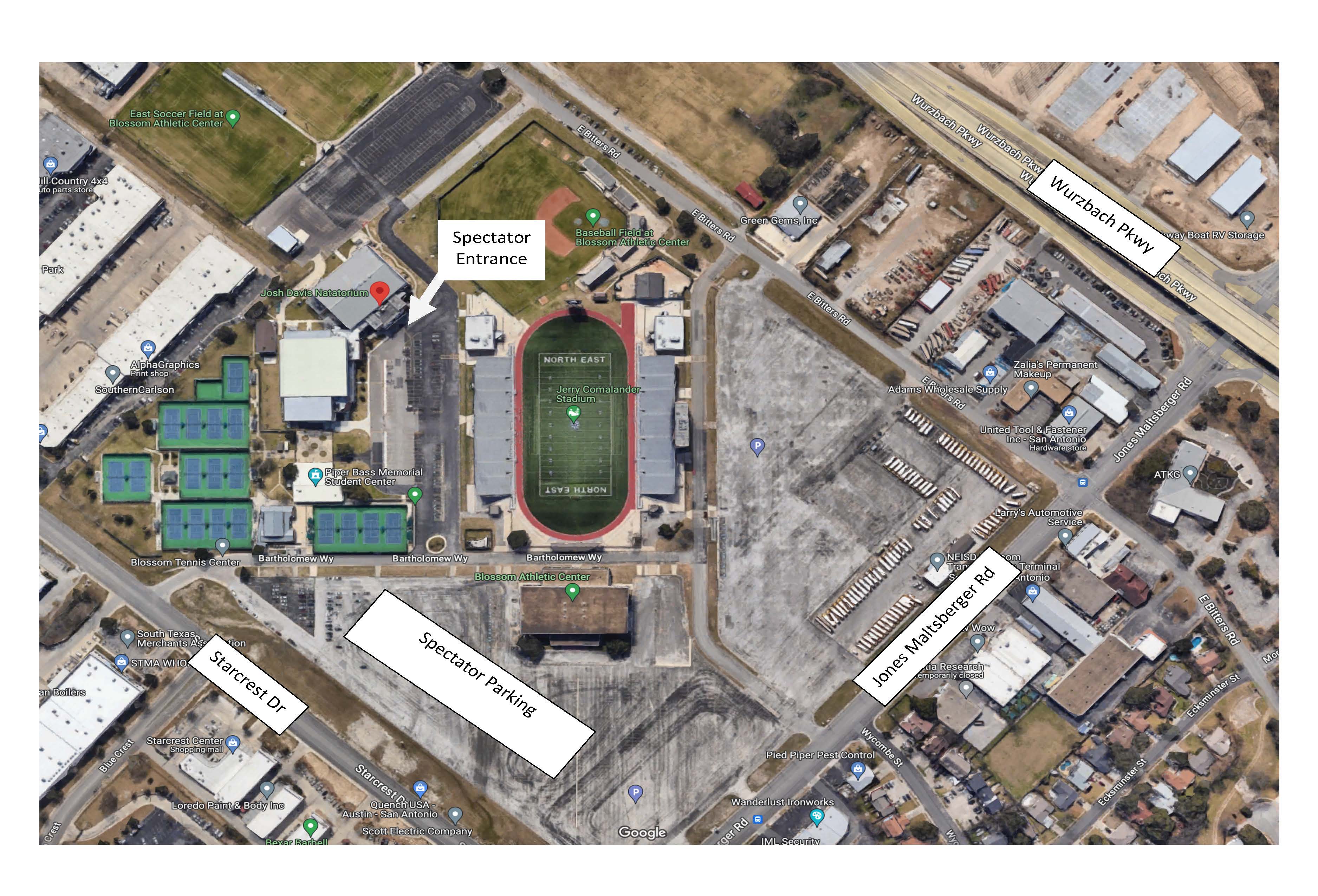The image is a detailed, high-altitude view, possibly from a drone or satellite, of a prominent sporting complex marked on Google Maps. Central to the image, slightly left of center, is the oval-shaped Jerry Comalander Stadium, identified by the distinct lines characteristic of a football field, with stands on either side and "northeast" labeled at both ends. Directly above this stadium lies the Baseball Field at Blossom Athletic Center. To the left of both fields, a hand-annotated note labeled "Spectator Entrance" points to a nearby parking lot and the entrance to the Josh Davis Natatorium. Additional labeled areas include the Piper Bass Memorial Center and a dedicated "Spectator Parking" area, emphasizing facilities for visitors arriving by car. Surrounding this complex are clearly marked streets like Woolsback Parkway, James Maltzberg Road, and Star Crest Drive, aiding navigation. Visible are various buildings, green fields, and infrastructural elements such as buses and rooftops, illustrating a comprehensive aerial perspective of the sporting area.